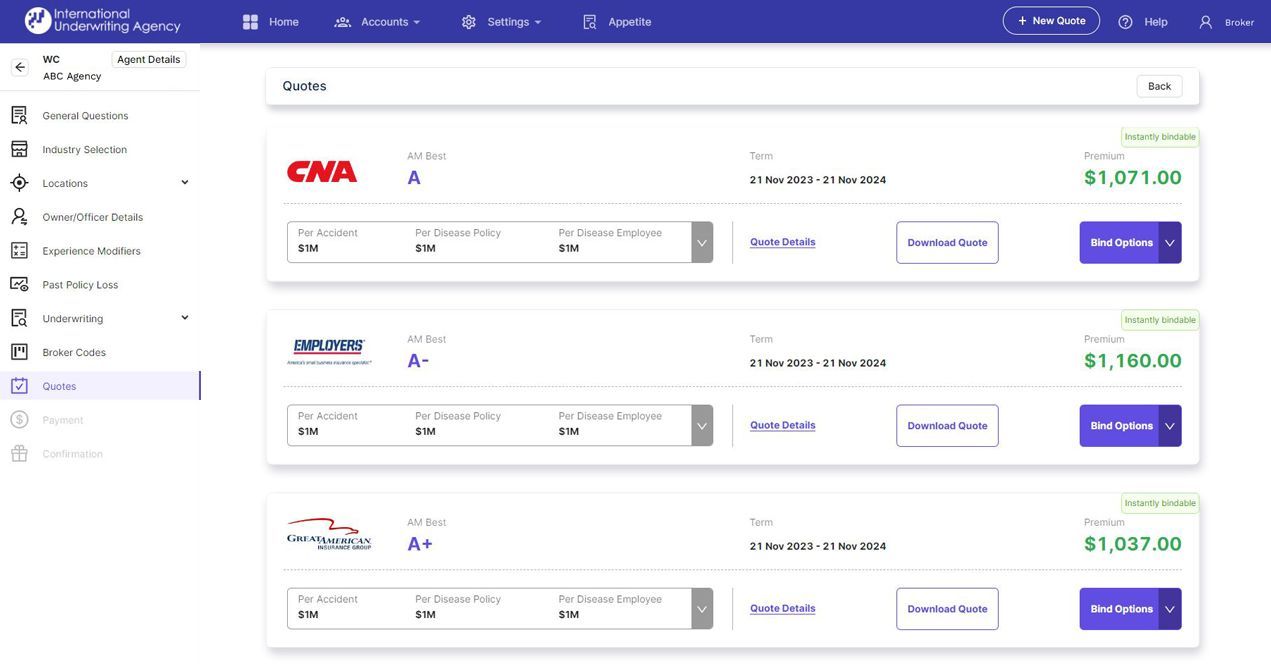The image displays a webpage screen on a computer with a stark white background and a top strip in dark royal blue. The top strip prominently features the title "International Underwriting Agency," indicating that the webpage belongs to some sort of insurance agency. Along this strip are menu options labeled "Home," "Accounts," "Settings," and "Appetite," accompanied by a small magnifying glass icon, likely representing a search function.

Directly beneath the blue strip, the text "WCABC Agency" is visible, alongside a small box labeled "Agent Details," suggesting that this is a personalized page for an agent tasked with creating quotes. On the far left-hand side of the screen, a vertical menu lists multiple navigation options including "General Questions," "Industry Selection," "Locations," "Owner Officer Details," "Past Policy Loss," "Underwriting," and "Broker Codes."

The central portion of the page showcases a range of insurance companies and policy types, complete with pricing information and AM Best ratings, presenting detailed descriptions of each policy. This detailed interface provides an agent with comprehensive tools for evaluating different insurance options.